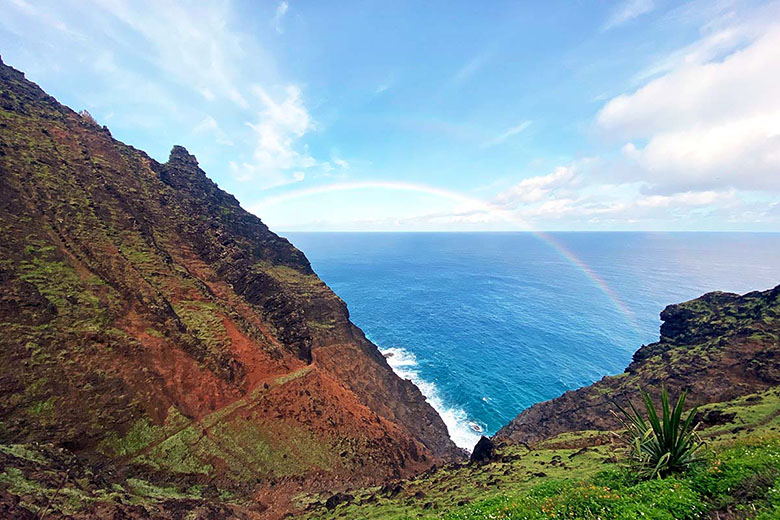This photograph captures a breathtaking daytime landscape from the vantage point of a cliffside, showcasing a rich interplay of natural elements. The foreground features rugged, jagged cliffs with a clay-like base softened by a lush layer of green vegetation. A narrow, winding trail is visible, cutting through the terrain and leading to a prominent V-shaped notch formed by another imposing cliff edge. At the base of these cliffs, the ocean begins, where the waves, whipped into white water, crash against the rocky shores.

Dominating the central portion of the image is a stunning rainbow, arching gracefully from the left side and seeming to touch both cliffs before disappearing into the sky. This rainbow serves as a captivating focal point, framed expertly by the photographer to enhance the visual drama of the scene.

The expanse of the ocean stretches out to the horizon, its surface a deep, serene blue, contrasting beautifully with the earthy tones of the cliffs and the vibrant greenery. Above, the sky is decorated with scattered white clouds that appear to be in motion, likely a result of a time-lapse effect, giving a sense of dynamic movement to the scene. The clouds seem to fan out from the horizon, blending seamlessly with patches of clear blue sky, adding depth and a sense of infinite space to this magnificent nature shot.